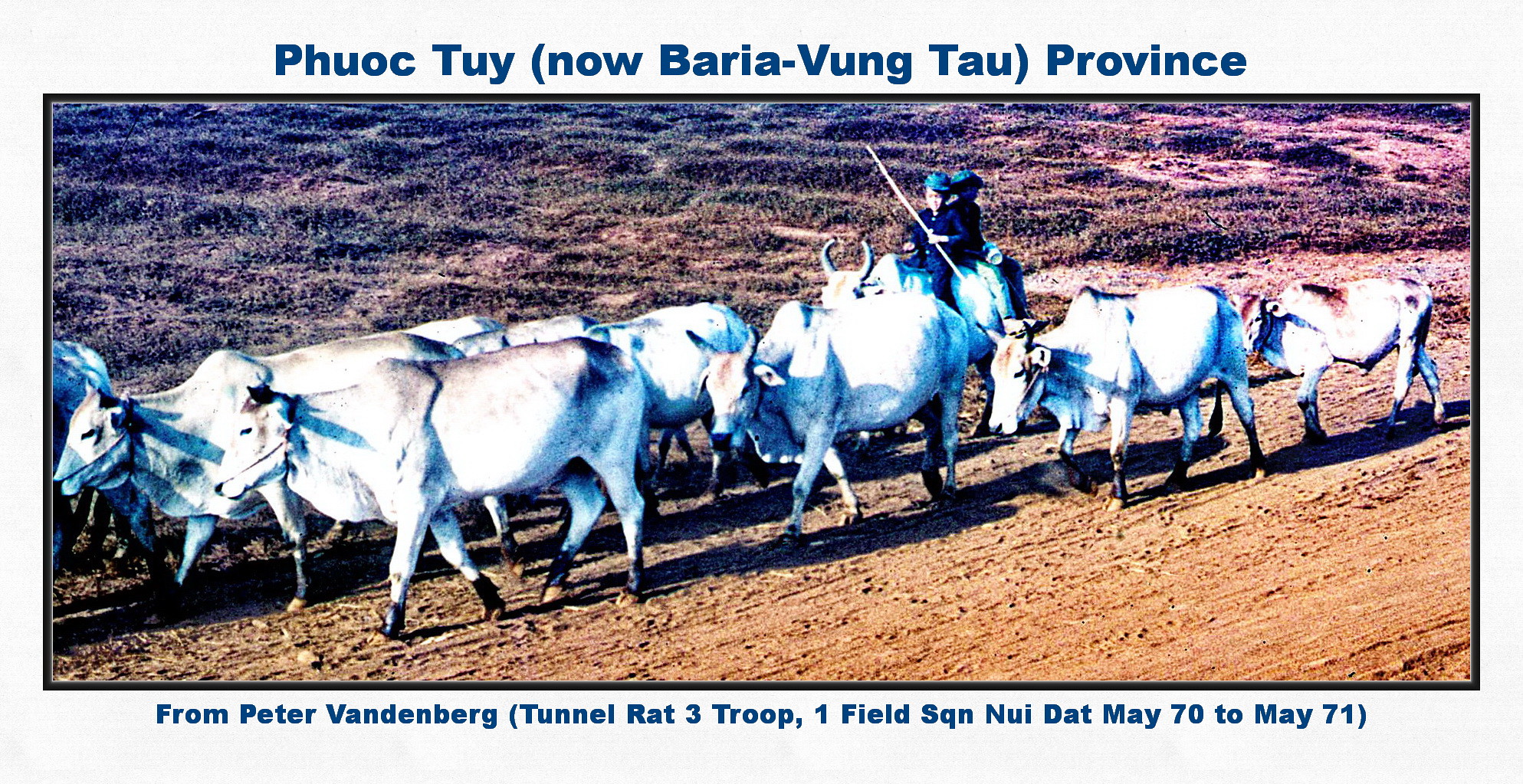This is an old, colorized photograph with blue-tinted text above it reading "Phuoc Thuy (now Baria Vung Tau Province)." The image features a row of white cattle, likely water buffalo, being herded by two boys wearing bucket hats and dark clothing. One of the boys is riding a buffalo, holding a long stick. The buffalo and their herders are walking along a mowed-down grassy area, which transitions to a rocky terrain with green grass in the background. The photo is adorned with a white banner, and text below reads "From Peter Vandenberg (Tunnel Rat Three Troop, One Field Squadron, Nui Dat, May 70 to May 71)." The overall aesthetic of the photo is aged and somewhat out of focus, contributing to its historical feel.